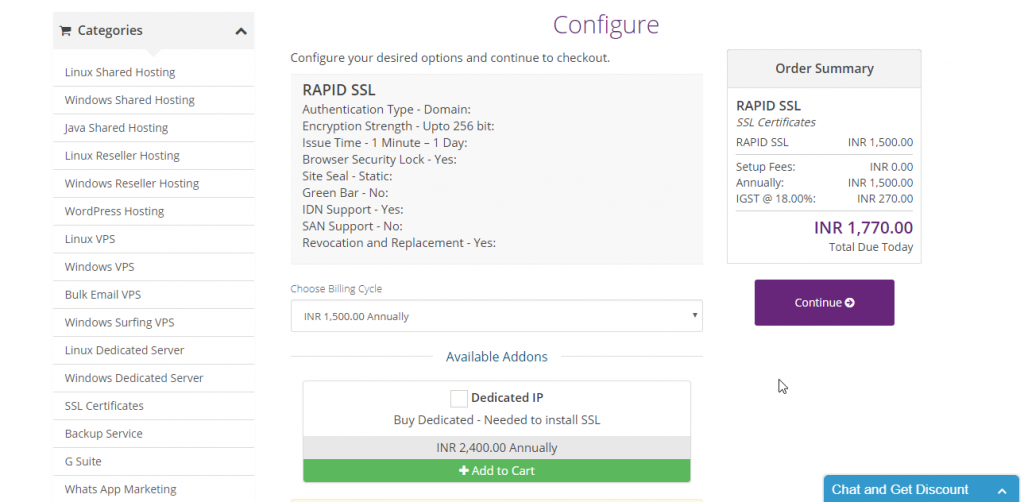This image depicts an order page from a website specializing in various hosting services. Dominating the upper left segment of the page is an expanded category dropdown menu, spanning the entire left side of the interface. This menu lists hosting options: starting with Linux Shared Hosting, Windows Shared Hosting, Java Shared Hosting, and extending further to include Linux Reseller Hosting, Windows Reseller Hosting, WordPress Hosting, among various other offerings.

At the top center, the heading "Configure" is prominently displayed, immediately followed by the instruction "Configure your desired options. Can you continue to check out?" The focus of this particular order is on RapidSSL, an authentication service for domains. Detailed specifications of RapidSSL are highlighted, showcasing encryption strength up to 256-bit, an issuance time between one minute to one day, browser security lock inclusion, a static site seal, but no green bar. Additionally, the service comes with ID and support but lacks SA and support. It does, however, include replication and replacement.

On the right side of the page, the order summary reveals that RapidSSL has been added to the cart with a total cost of INR 1,770. The acronym INR denotes the currency in Indian Rupees. Below this summary, a prominent purple "Continue" button invites the customer to proceed with their transaction.